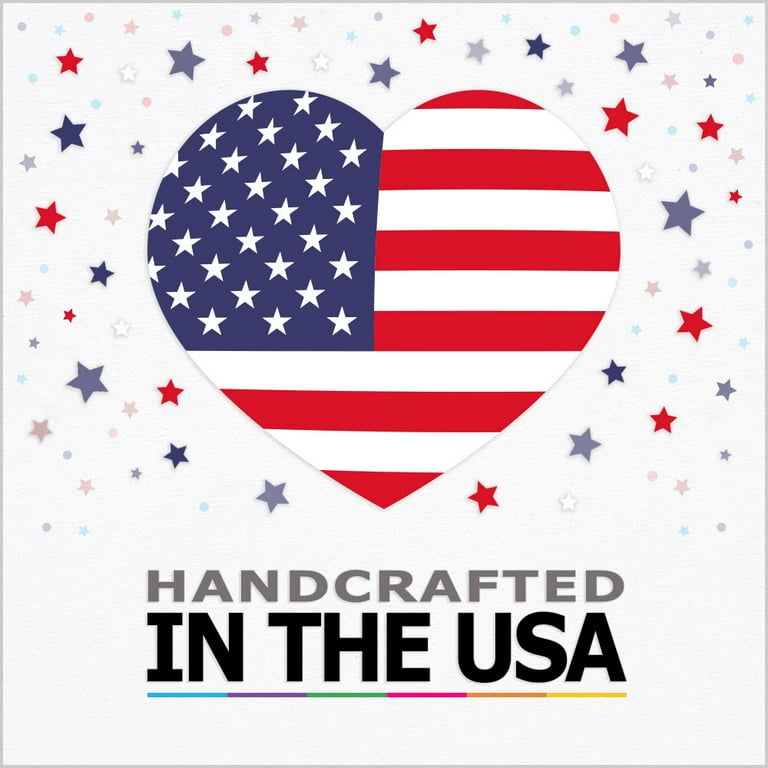The image depicts a white poster with a central heart design that incorporates the American flag. The heart features the blue field with white stars in the upper left portion and red and white stripes filling the rest. Surrounding the heart are numerous colorful stars in shades of turquoise blue, navy blue, red, dark grayish-red, and pink, along with various colorful dots. The stars and dots vary in size, creating a dynamic background. At the bottom of the image, the text "Handcrafted" appears in gray capital letters, followed by "in the USA" in black text. Beneath this text is a thin, rainbow-colored stripe featuring segments of blue, purple, green, pink, orange, and yellow. The entire design rests on a white background with a slight papery texture and is framed by a light blue border.